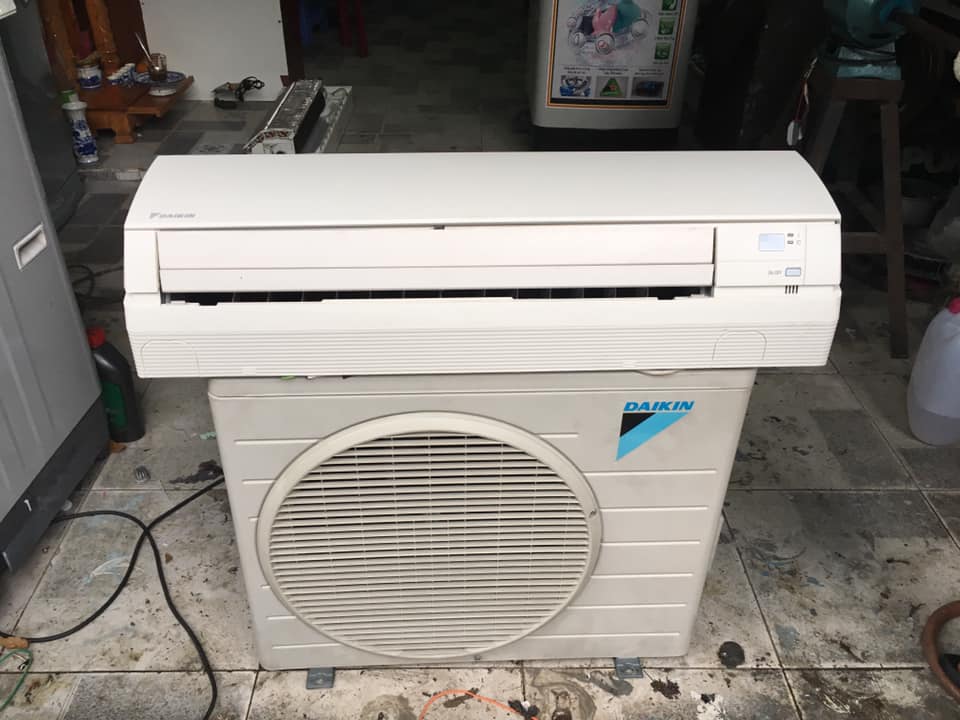Inside a dimly lit laundry room with a cluttered, marble-patterned gray and light gray tiled floor, sits a cream-colored Daikin air conditioning unit. The distinctive Daikin logo, consisting of the name "D-A-I-K-I-N" in blue letters alongside a blue and black triangle, is prominently displayed on the upper right corner of the equipment's base, which features a circular vent. Stacked atop this square unit is a smaller, rectangular component, somewhat resembling a printer or fax machine, sharing the same light beige hue. Scattered on the floor to the left is a black power cord. Surrounding the equipment, a gray closet door with a white handle is visible on the far left, while a wood shelf with vases and a wooden tripod peek out from the upper left and right corners, respectively, adding to the room's utilitarian yet homey atmosphere.